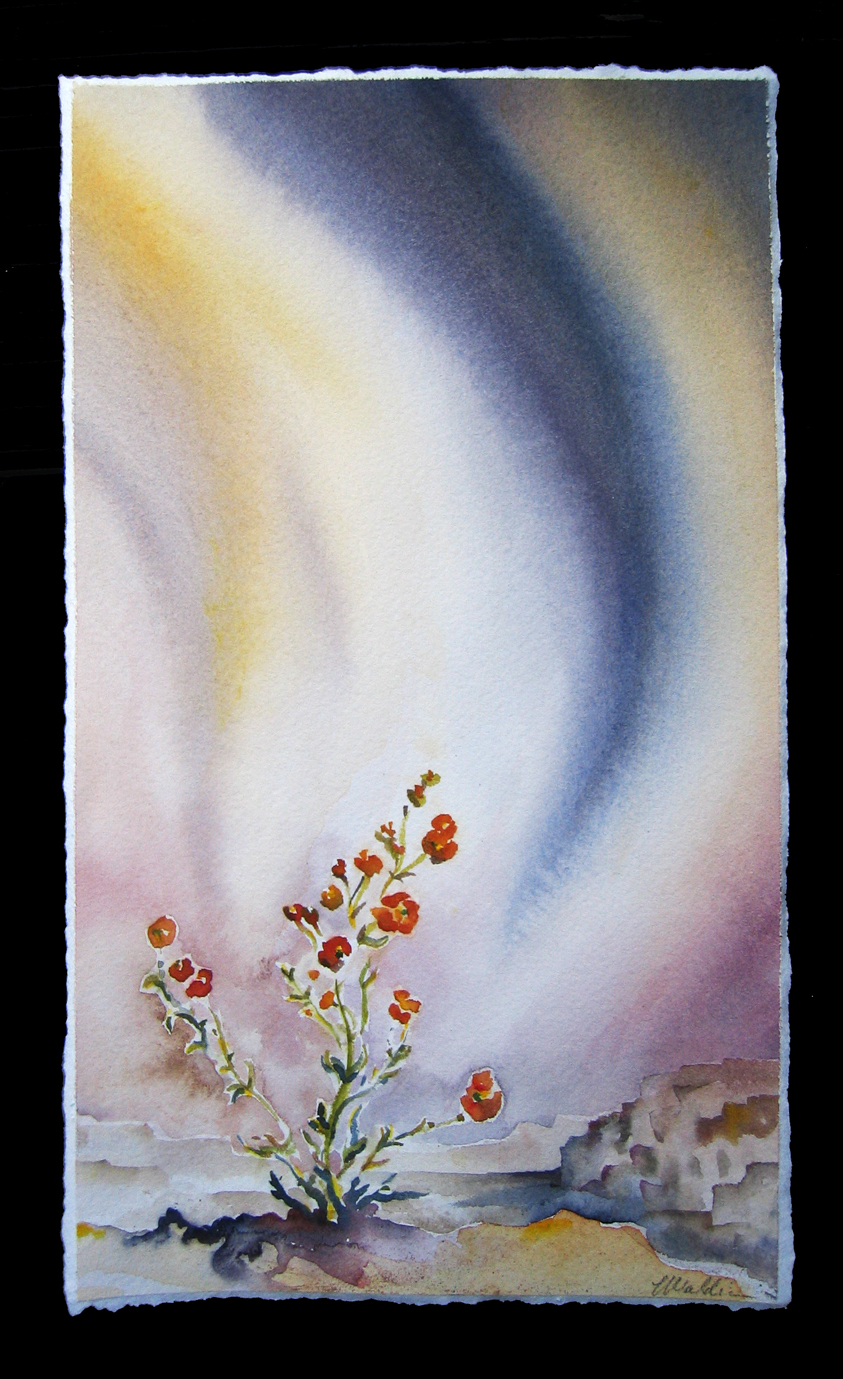The image is a vibrant framed watercolor painting with a thick black border. The background features an abstract wave of colors transitioning from blue, dark blue, orange, yellow, and white at the top, blending into shades of purple and dark pink towards the bottom. In the foreground, on the bottom left, a green plant with a sturdy green stem and several red flowers edged in orange blooms out of bluish-brown earth. The plant has about 15 to 20 flowers and lush green leaves. On the bottom right, partially depicted, is a small village with not very clearly drawn houses, one of which is a white house with a brown roof. The sky contains colorful shapes reminiscent of Toledo tails, with the left side primarily yellow and the right side predominantly blue. The overall composition is detailed, blending various hues and shapes to create a harmonious, picturesque scene.